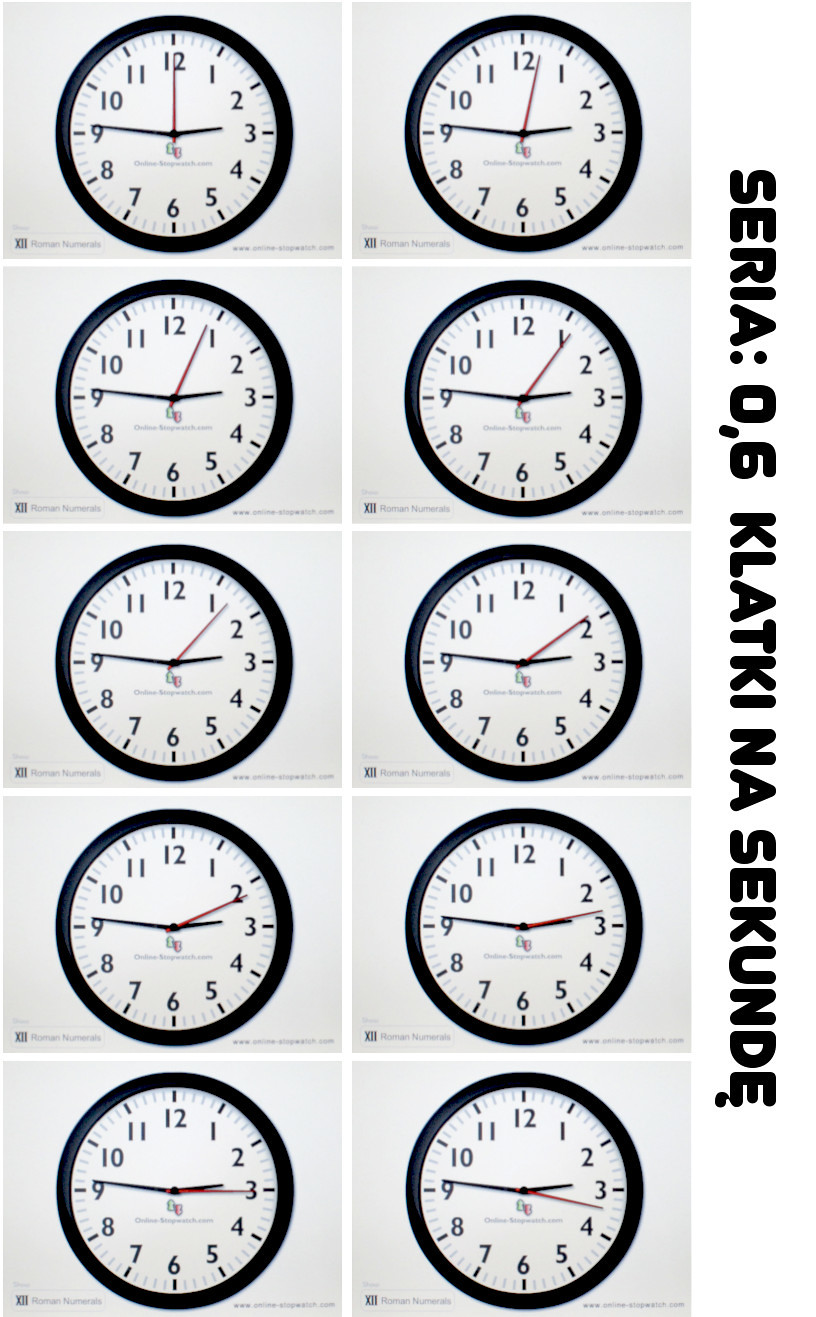The image is a color graphic featuring 10 round clocks, arranged in two columns and five rows, each clock set at 2:45 but differing slightly with each second hand position. The clocks have a black border, a white face, black numbers, two black hands, and a red second hand. The background is consistently white. Along the right side of the series of clocks, there is text in a foreign language that reads "S-E-R-I-A, colon, 0.6, K-L-A-T-K-I-N-A, S-E-K-U-N-D-E" in a vertical orientation. The image is much taller than it is wide, with no people present in it.